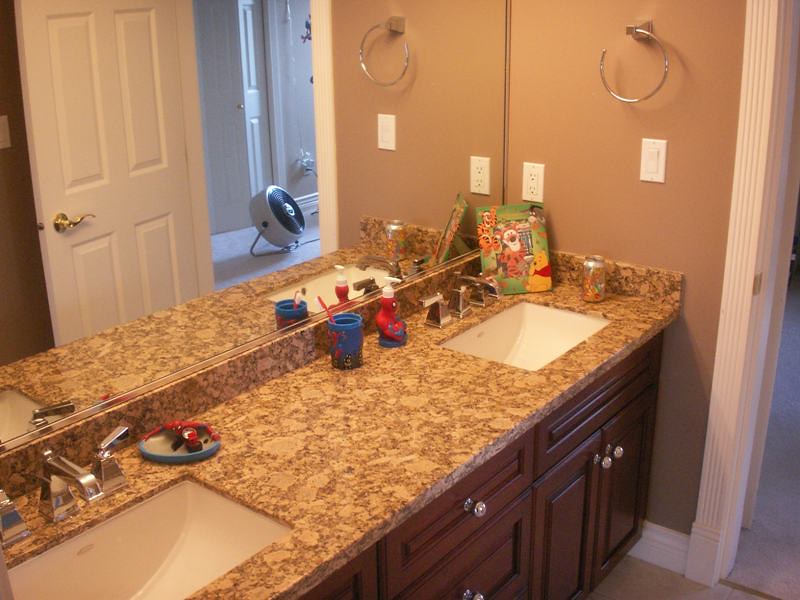The photograph captures the interior of a bathroom with distinctive features and a view into an adjoining carpeted room through an open door adorned with white trim and a gold-colored handle. The taupe-colored bathroom walls are complemented by dark brown cabinets and a speckled brown countertop, which has an elegant double-sink setup with square-shaped basins. Both sinks feature square-ish silver faucets. Hanging on the wall is an almost complete silver circle, likely serving as a towel holder.

In the reflection of the bathroom mirror, the carpeted room is further revealed, where a circular floor fan is visible. Adding a touch of whimsy, a picture of Tigger, Winnie the Pooh, and Eeyore is positioned in the corner of the bathroom, near the mirror. An aluminum can with indistinguishable colors sits on the countertop alongside a Spider-Man themed soap dispenser, a blue cup with a red toothbrush, and a circular item featuring a crouched Spider-Man holding a blue edge. This image highlights the bathroom's blend of practical elements with playful, character-themed accents.